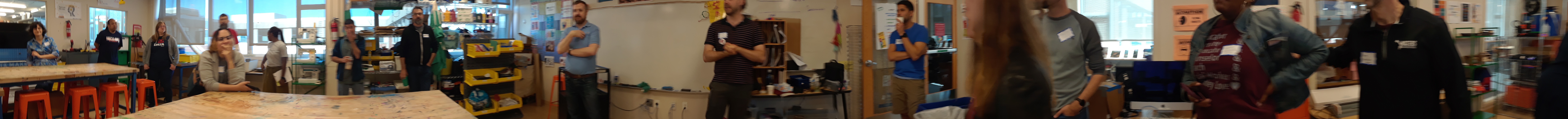The image is a narrow, panorama-style snapshot of an active workshop or classroom setting. The left side of the image showcases a background wall lined with plate glass windows in front of which stand steel shelves filled with numerous boxes and bins. In the foreground on this side is a large piece of plywood. There are several people, about eight, facing the camera as if posing for a photograph. Moving to the center, the background transitions to a tan wall where more individuals, mostly males, are also posing for the camera. To the right, the image partially captures three individuals from the chest down to the waist with their heads and legs out of the frame. They are in front of light-colored walls and more plate glass windows with bins and racks for storage. Some people have white name badges on their left breast area, indicating a formal or organized setting. Scattered throughout are wooden shelves, red chairs, desks, and a wooden table or desk. A female with dark hair is seen sitting at the furthest left while another female is by herself at a middle table. The scene also includes a whiteboard on the right side, in front of which two people are possibly instructing. The overall impression suggests a vibrant learning space or workshop bustling with activity and populated by a diverse group, predominately male, and equipped with various teaching and storage materials.